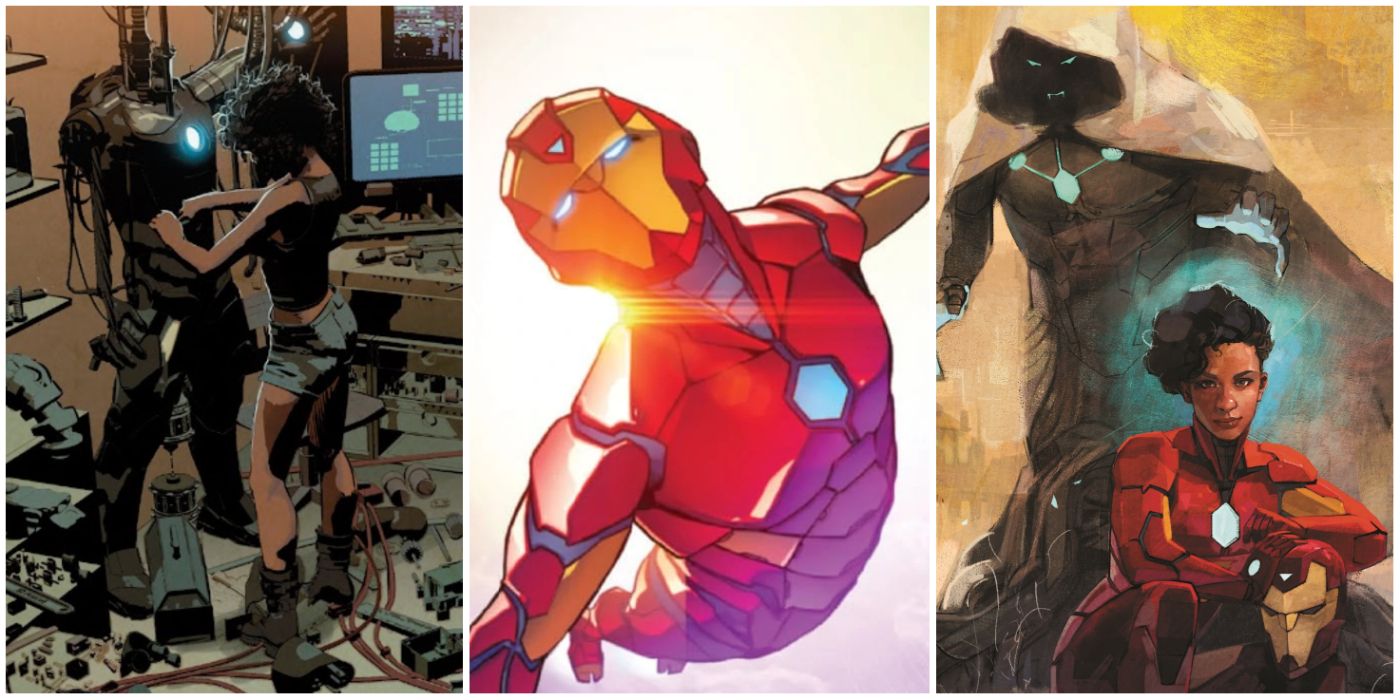The image is a triptych of illustrations from a Marvel Comics series featuring Ironheart, a young African American woman who wears a suit resembling Iron Man's armor. 

In the first image on the left, she is in a dimly lit workshop or computer lab, assembling the Ironheart suit. She is dressed in a tank top, shorts, and boots, surrounded by tans, browns, and blacks, with a bright light emanating from the suit's chest and a computer screen providing additional illumination.

The center image depicts Ironheart soaring through the air with the sun gleaming behind her shoulder. The suit is predominantly red with a blue abdomen and features a glowing octagonal port on the chest and illuminated eyes. The helmet has a golden-red hue, enhancing the impression of her flying.

The third image shows Ironheart sitting on the ground, holding her helmet between her knees, with her elbow resting on her legs. She is in a moment of apparent vulnerability as a menacing villain looms behind her. The villain, clad in a hooded cape, also has multiple glowing areas on his suit, matching Ironheart's design. His fangs and eyes are illuminated, and an ominous blue light radiates around her head from his outstretched hands.